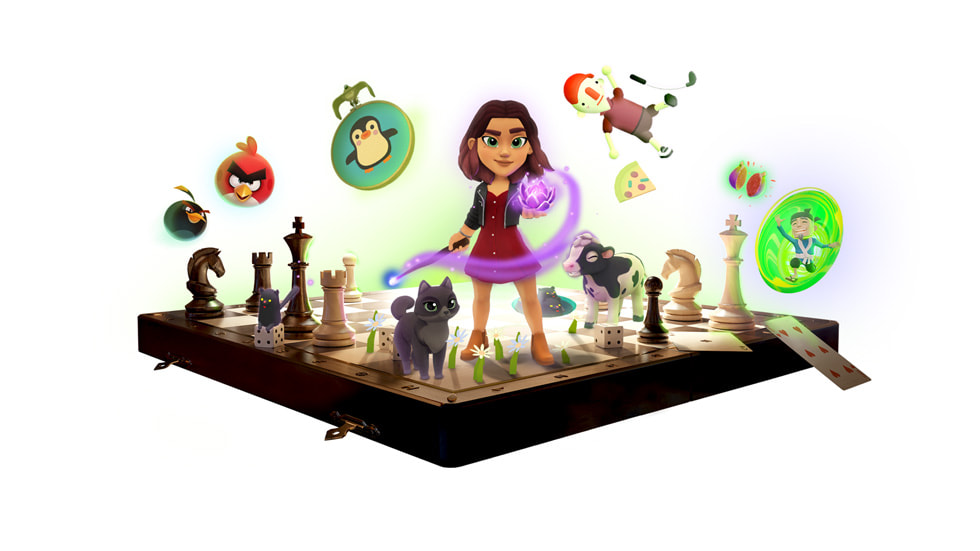In this detailed and vibrant illustration, a variety of iconic video game characters and elements are depicted standing on a large chessboard. The central figure is a female cartoon character, holding a wand in one hand and a mystical orb emitting a purple glow in the other. Her calm, poised demeanor contrasts with the playful chaos surrounding her.

To her left is a black cat with piercing green eyes, adding an air of mystery. Behind her, chess pieces, both black and white, are scattered, creating a classic yet whimsical backdrop. Notable characters include the animated, mischievous Angry Birds—a red bird and the black bomb bird—floating above the chessboard with playful intensity.

On the left edge of the chessboard, a knight and rook chess pieces stand prominently beneath the Angry Birds. Adjacent to the central figure, a peculiar floating medallion showcases a penguin inside it, and a skateboarder attempts a flip, humorously captured as a pizza slice slips from his grasp. Below, a cow nonchalantly stands on the chessboard, adding a surreal touch.

On the right, we see references to mobile games with the presence of a Fruit Ninja character, further accompanied by random elements such as playing cards, dice, and flowers intricately placed within the scene. The ensemble creates a dynamic, fantastical world blending various gaming universes into a single captivating image.